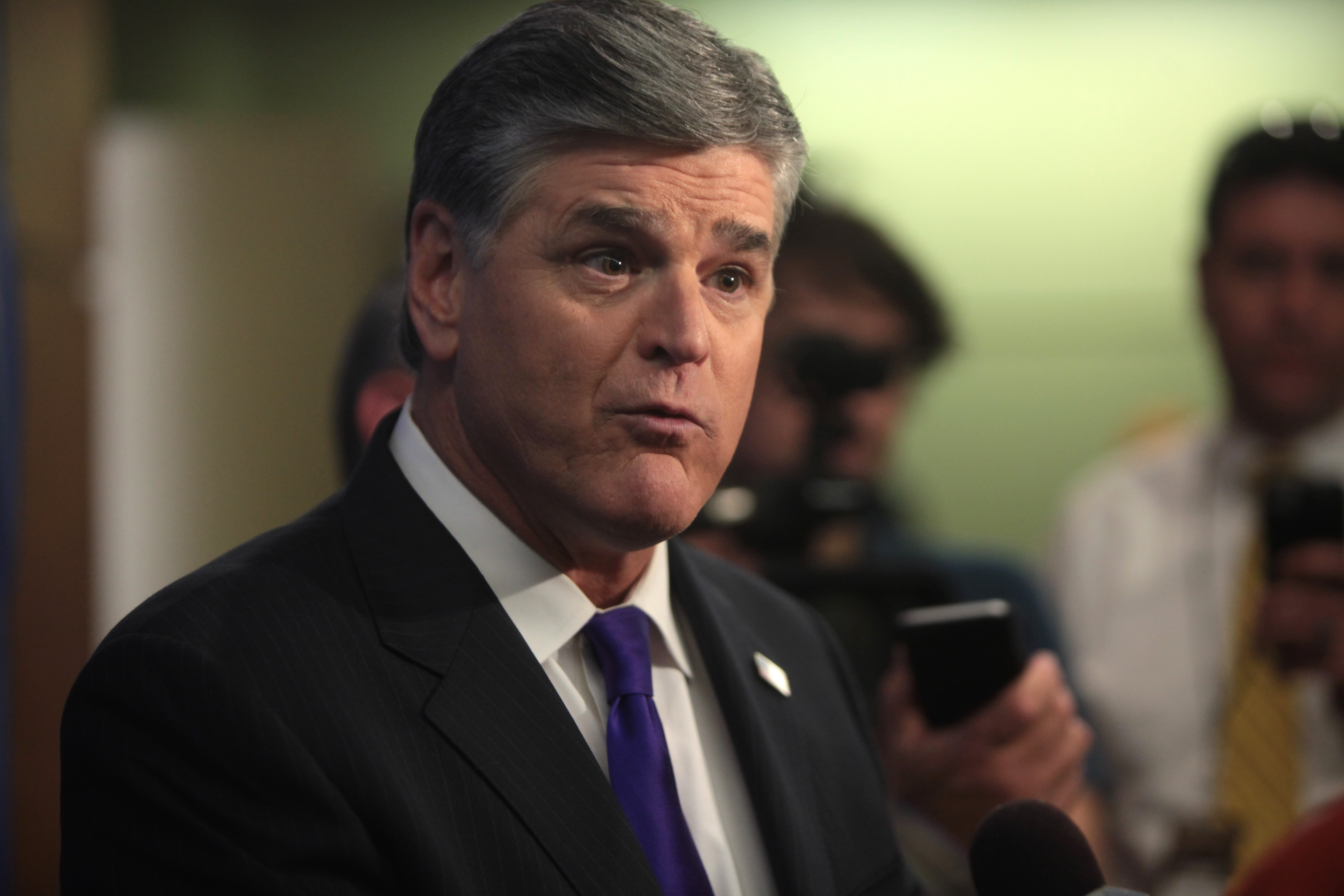The photograph, horizontally aligned and rectangular, showcases a man in the foreground, possibly the Fox News host Sean Hannity. He is dressed in a black suit jacket, a white button-down shirt, and a vibrant purple tie, adorned with a lapel pin on his left chest. The image captures from his chest up, highlighting his slightly open mouth as if he is speaking, and his raised eyebrows which create wrinkles on his forehead. His grayish-white, wavy hair is neatly combed, and his brown eyes are directed to the right. 

In the blurred background, there are several other individuals, likely reporters, including one holding a camera up to their eye and another with a cell phone in hand. These figures are indistinct, bringing the primary focus onto the man at the center. Below him, to the bottom right, a microphone is partially visible. The overall backdrop features a mix of blurry whitish-green hues, possibly influenced by lighting, with elements of brown on the left side.